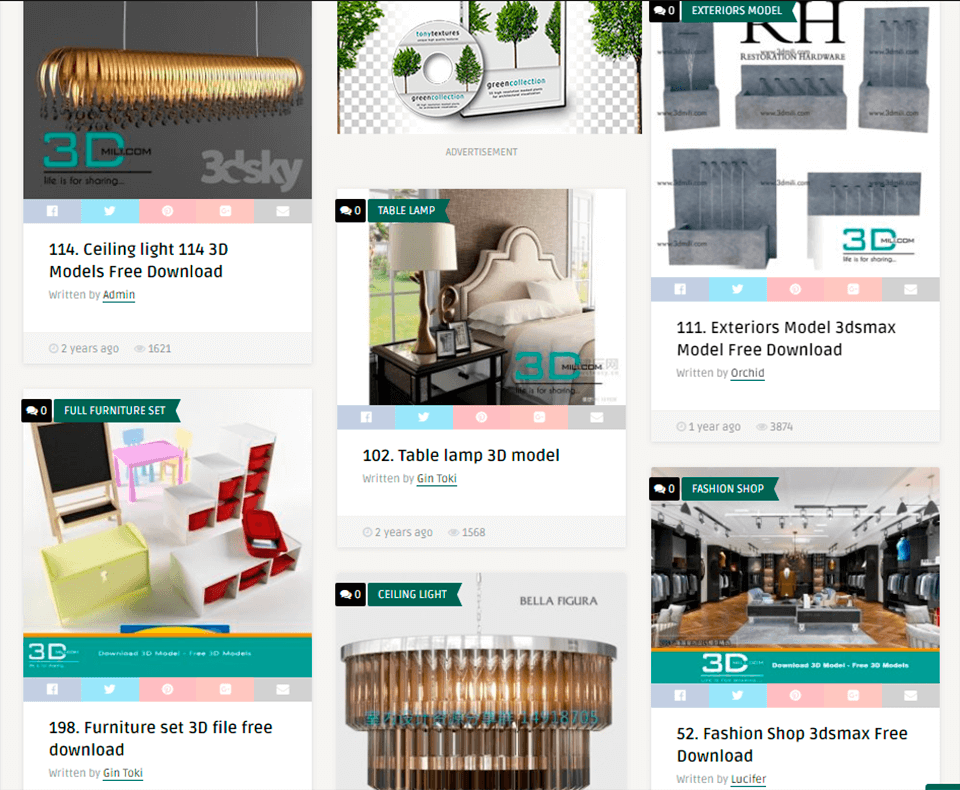The image is a collage of social media screenshots that showcase various 3D models available for free download. The top-left section features an intricately designed golden object with grooves along its sides, labeled "114 Ceiling Light," hinting at its availability in three different 3D models. Below this, an advertisement for a child’s bedroom playset is displayed, which includes a wooden chest, a desk with drawers, and a small table that resembles a TV stand, marked as "138 or 198 Furniture Set 3D File Free Download." In the top-middle section, another advertisement is present featuring a CD and a CD case adorned with tree graphics. Below this, a bedside setup is portrayed, complete with a table, a lamp, a bed, and two pillows, described as a "102 Table Lamp 3D Model." Finally, on the right side of the image, there is a reference to an exterior model labeled "111 Exterior Model 3D Max Model Free Download."